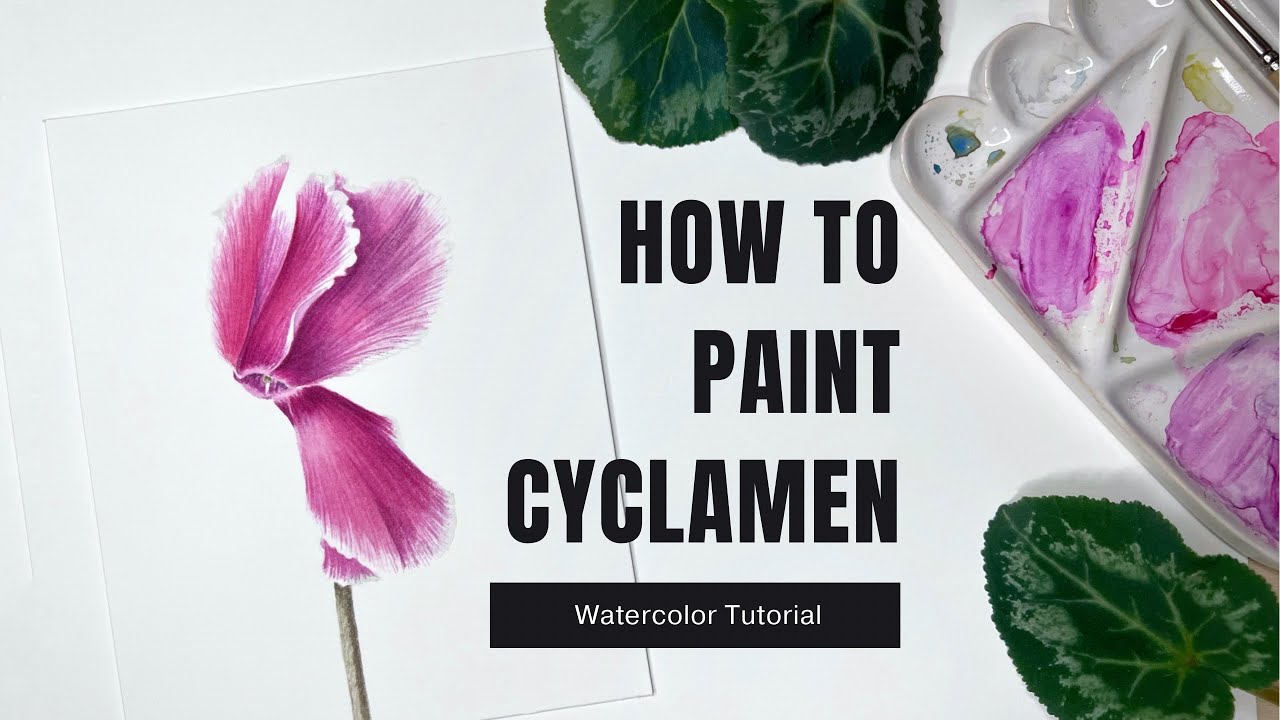The image showcases a detailed introductory scene for a watercolor painting tutorial titled "How to Paint Cyclamen," prominently displayed in bold black sans-serif text on a white background. Beneath this title, a small black box contains the subtitle "Watercolor Tutorial" in white text. The center of the image features a realistically painted cyclamen flower on a slightly askew white paper. The flower has delicate pink petals with white-lined edges that stretch upwards and to the right, as well as downwards. A brown stem emerges from behind the petals, leading to two detailed green leaves with white veins—one larger leaf at the top and a smaller one at the bottom right of the frame. To the top right of the image, there's a white, scalloped dish palette with triangular compartments that hold pink smudges of watercolor paint, indicating the colors used for the artwork. This setup, complete with the realistic flower depiction, green leaves, and the artist's palette, encapsulates a serene and instructive scene aimed at guiding viewers in painting cyclamen flowers with watercolors.